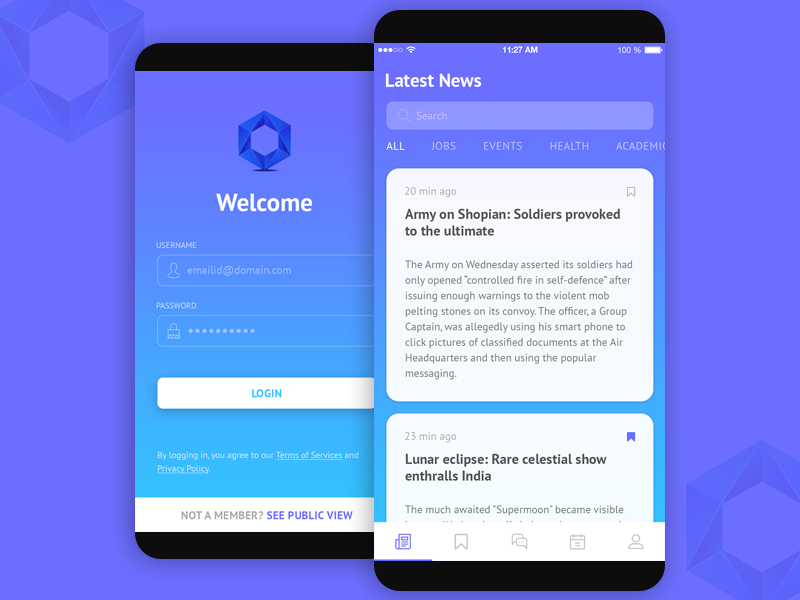The image depicts a login screen against a blue polygonal background that resembles a hexagon. The top left and bottom right corners display the word "Welcome" within the hexagonal shape. The login form features fields labeled "User" and "Email ID," with a sample email "emailid@domain.com" provided as a placeholder. A password field shows approximately ten concealed characters. Below the fields, there's a "Login" button followed by a disclaimer stating, "By logging in, you agree to our terms and services and privacy policies." At the bottom, a note reads, "Not a member? See a public view."

Adjacent to this is another screen displaying various indicators and sections. At the top, icons indicate full WiFi signal strength, the time (11:27 AM), and a 100% battery charge. Below these icons, there are three filled circles and two unfilled ones. The middle section highlights the "Latest News" with a search bar and tabs labeled "All," "Job," "Events," "Health," and "Academics" for sorting content.